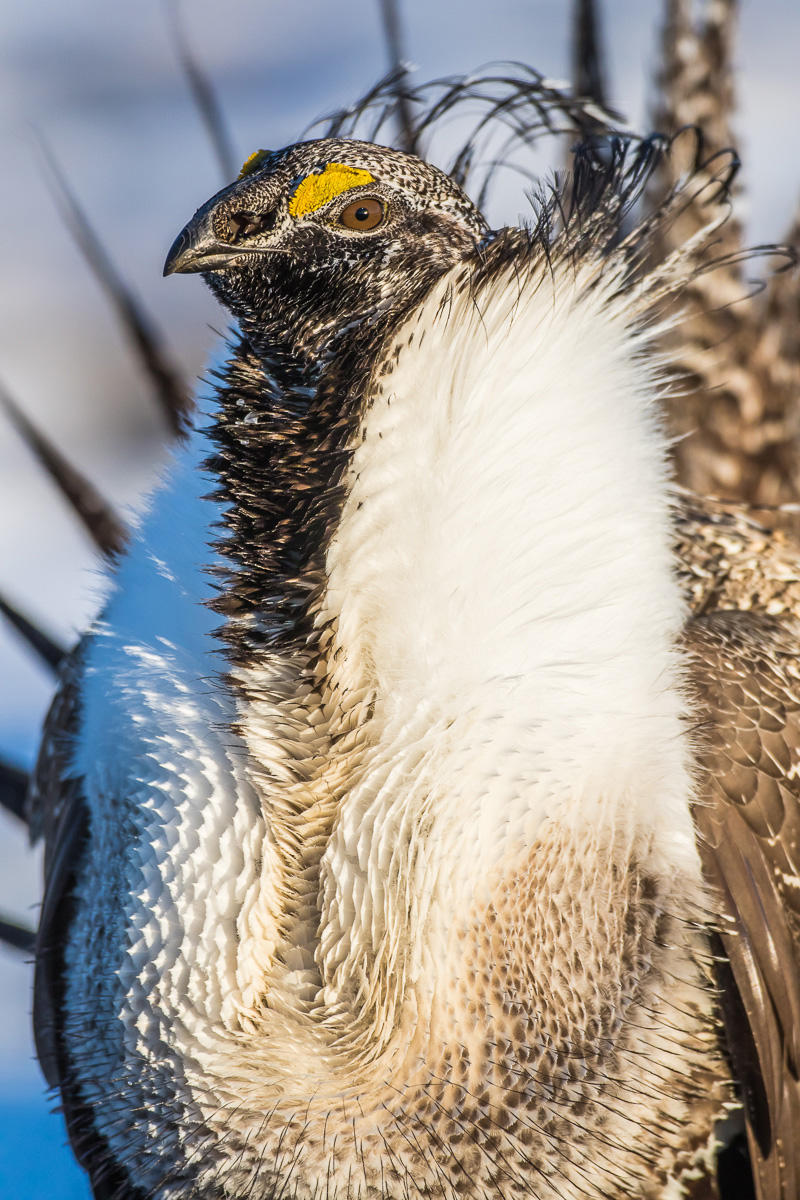This close-up photograph, taken outdoors in daylight, showcases a detailed view of a turkey with striking features. The bird's black beak stands out against its predominantly black and white mottled face. It has distinctive yellow eyelids and a prominent orange mark above its light brown eye with a black pupil, giving it a striking appearance. The turkey's thick, puffy white feathers cover its breast, which transitions to brown towards the bottom. The neck appears black while long, thin, black and white feathers sprout from the back of its head, giving a slightly spiky impression, and the background is blurred, focusing on the bird. Additionally, the bird's large tail feathers, visibly pointing to the left and out of focus, along with a mix of brown and white feathers, can be seen behind its breast. The sun illuminates the scene, accentuating the bird's vivid details against the blue sky dotted with scattered white clouds, creating a compelling and natural portrait without any text.